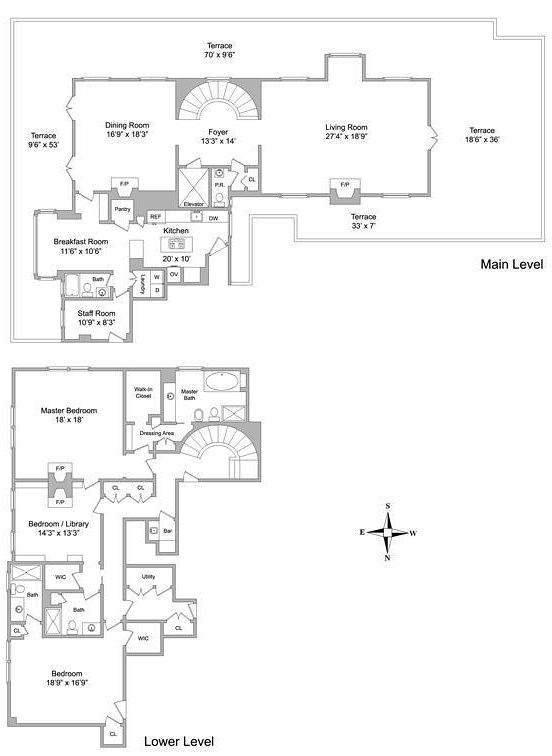This image features a detailed blueprint of a house layout, showcasing both the main and lower levels. The blueprint is rendered in various shades of grey and small black text, laid out in a clear and organized manner across a standard page size.

The main level spans the top half of the page, with distinct rooms and dimensions marked. Dominating the left side is a slightly L-shaped terrace, with the longer part of the "L" oriented horizontally. Adjacent to the terrace, the dining room is indicated, measuring 6.9 by 18.3 units. The foyer and living room extend centrally, leading out to another terrace on the opposite side.

The lower level is positioned towards the bottom of the blueprint, directly showing the layout of the bedrooms. This floor comprises three bedrooms, emphasizing the residential nature of the house. Additionally, a compass rose in the lower right corner provides orientation with north, south, east, and west directions clearly marked.

Overall, the blueprint is simplistic yet detailed, offering a comprehensive view of the house's structure in a monochromatic scheme.